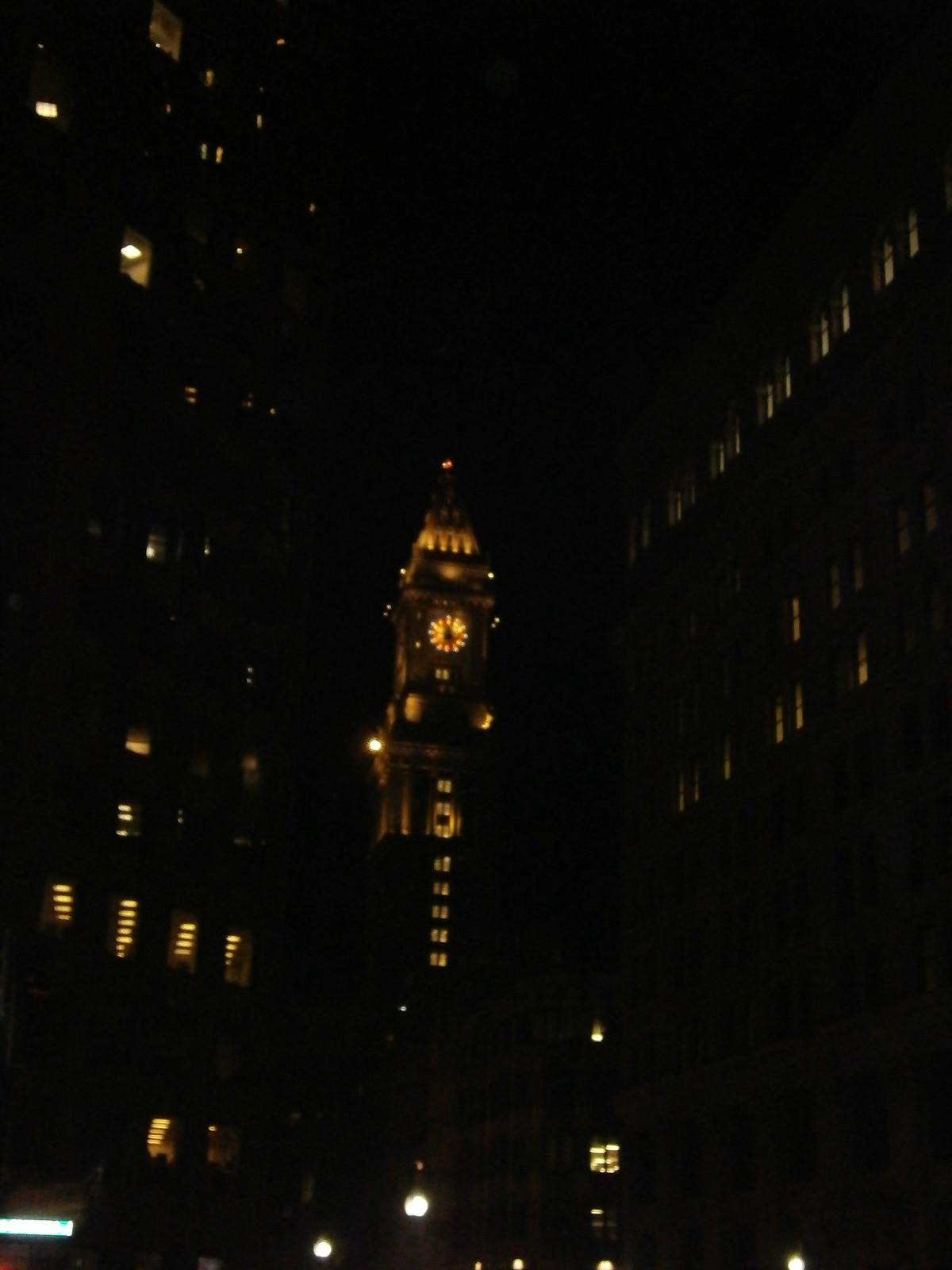This nighttime photograph captures a cityscape from ground level, looking upwards. Dominating the center of the image is a tall, pointed tower reminiscent of a clock tower, though it is not Big Ben. The tower’s clock face is illuminated, casting a gentle glow against the pitch-black sky. The surrounding buildings flank both sides of the tower, with several windows emitting light, indicating some occupancy despite the late hour. Streetlights and other scattered lights visible at ground level add subtle brightness to the dark scene. The stark contrast between the illuminated architectural elements and the dark surroundings gives the image a dramatic, almost serene quality, with no stars visible likely due to the camera's focus on the urban features.